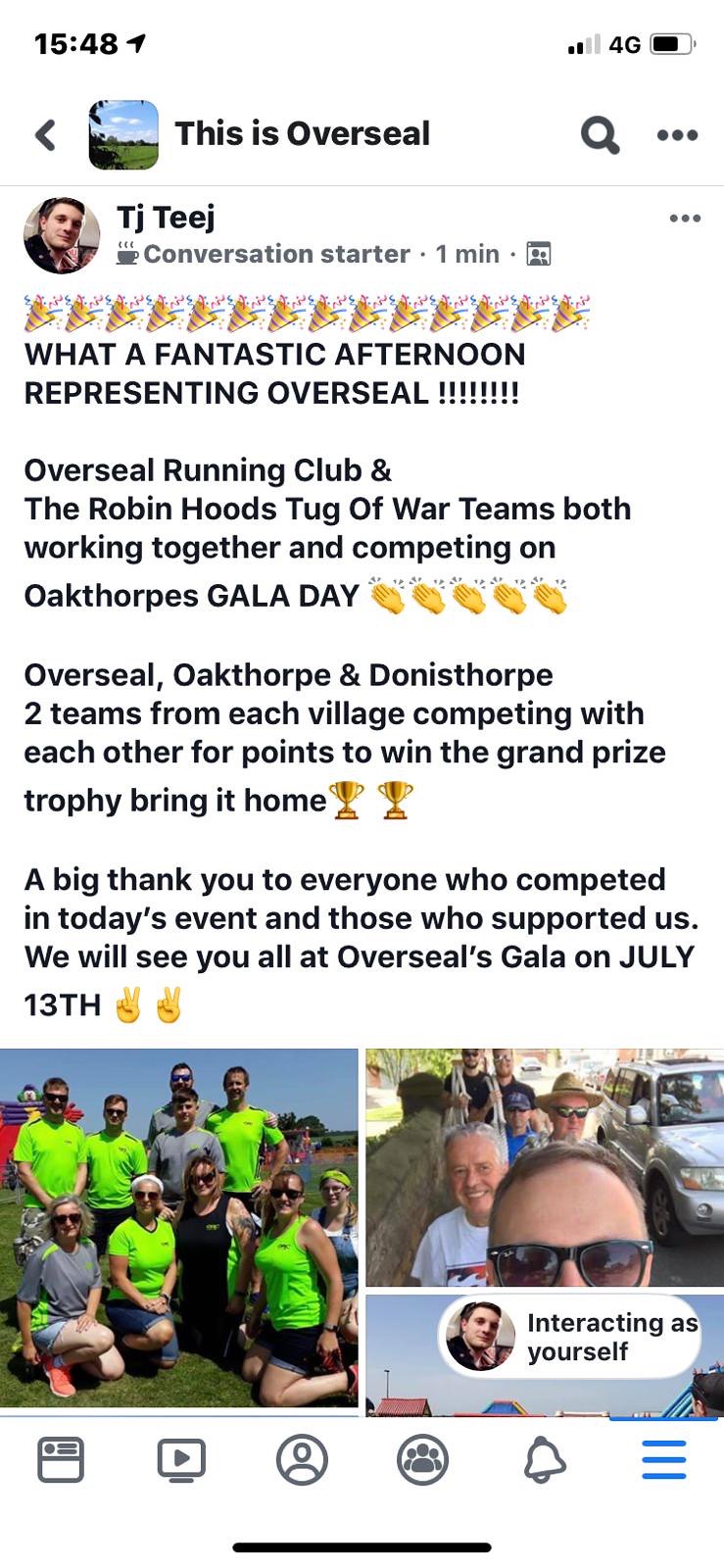The image is a detailed screenshot of an Instagram post titled "This is Overseal" by user TJ Teague, labeled as a "Conversation Starter." The phone displays the time 15:48, and the status bar shows two out of four signal bars, 4G connectivity, and a battery that's a little more than half full. At the top of the screen, navigation icons such as a back button, a search icon, and a menu with three dots are visible.

The post celebrates a wonderful afternoon representing Overseal, featuring the Overseal Running Club and the Robin Hood Stagger teams. These teams, from the villages of Overseal, Oaks Thorpe, and Donna's Thorpe, participated in friendly competition during Oaks Thorpe's Gala Day. The objective was to accumulate points and win the grand prize trophy. The post includes a clapping emoji and a trophy emoji to emphasize the excitement and gratitude towards everyone who participated and supported the event. The announcement concludes with a note about the next event, Overseal's Gala on July 13th.

Below the text, there are two images: one on the left and one on the right. The left image shows a group of older adults wearing bright green and gray jerseys, posing for a group photo. The right image is a selfie with the same group of people, all smiling. The Instagram interface icons are visible at the bottom of the screen.